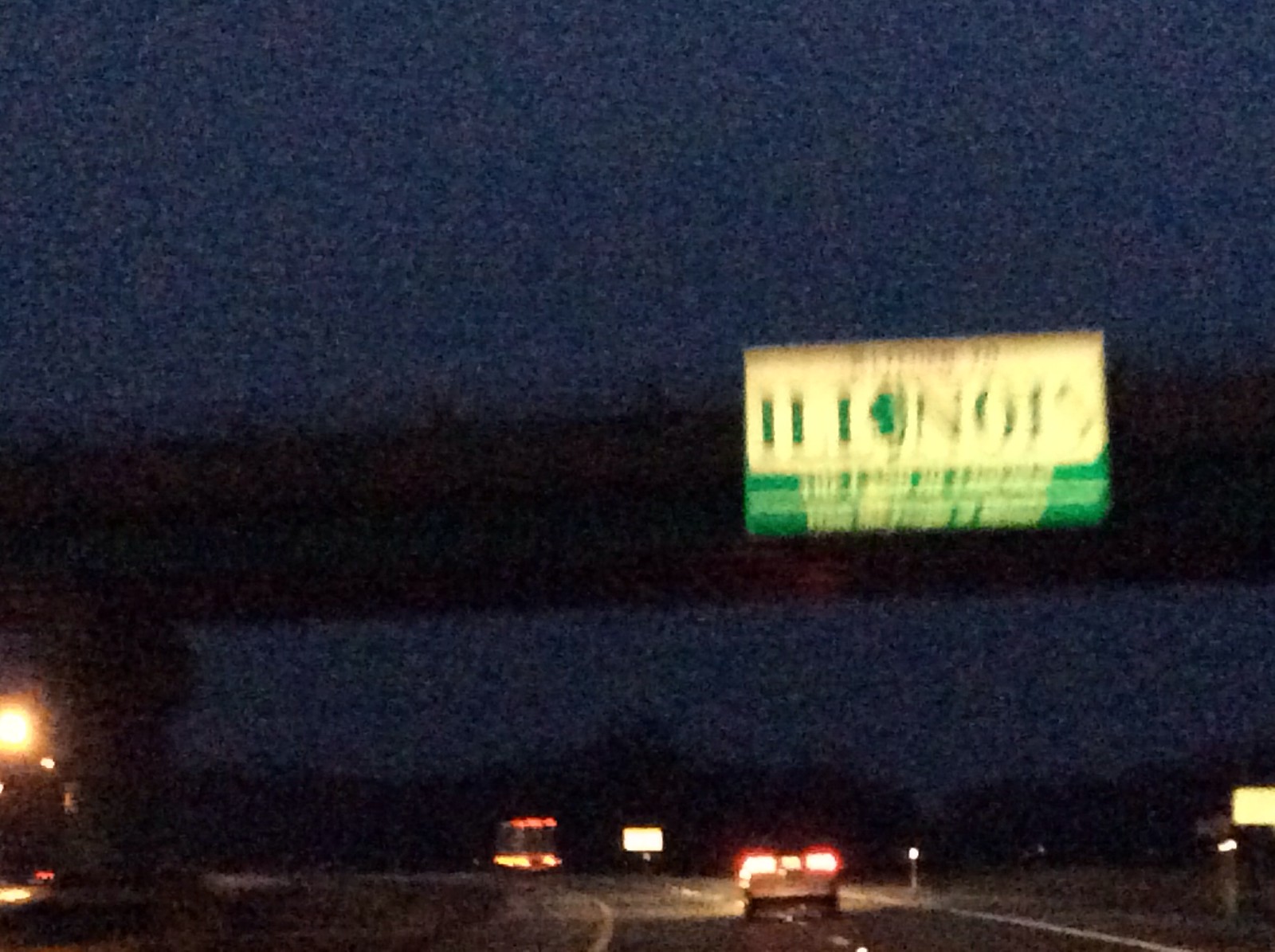A blurry, low-resolution nighttime photograph captures a highway scene from inside a car. In the foreground, two vehicles are visible on the road ahead. The one furthest ahead seems to be a bus, while the nearer one appears to be a typical sedan. The scene features an overpass or bridge crossing above the highway, with a green and white illuminated sign attached to it. However, due to the blur, the text on the sign remains indecipherable, allowing only the colors to be distinguished. The darkness and motion blur add a sense of movement and fleeting visibility to the scene.